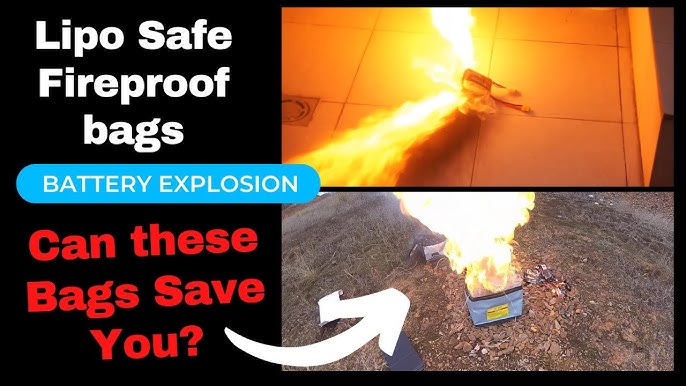The image is an advertisement for LiPo Safe Fireproof Bags, showcasing their effectiveness in containing battery explosions. On the left side, white and red text reads "LiPo Safe Fireproof Bags" and "Battery Explosion," followed by the question "Can these bags save you?" highlighted in blue and red. The advertisement features two photographs: The top one is an informal, home-taken image of a LiPo battery explosively catching fire indoors on a tiled floor, with flames shooting out from both sides and a drain visible on the left. The bottom photograph, taken outdoors on a pile of rocks surrounded by dirt, shows a LiPo battery contained within a fireproof bag, with the flames directed upwards, contained more safely. A prominent white arrow points to the bag in the second picture, emphasizing the difference in fire behavior when the battery is protected by the bag.